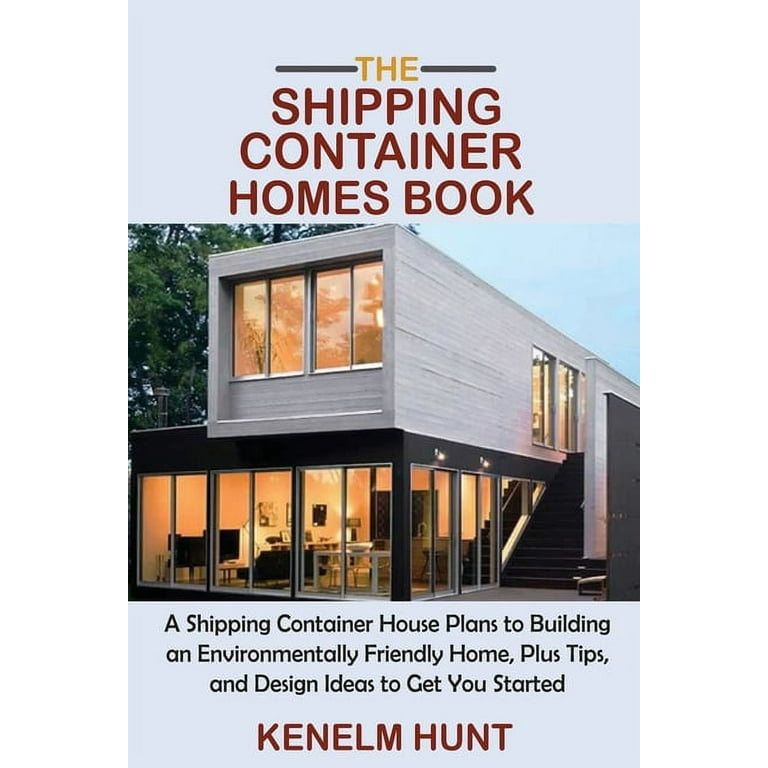The cover of "The Shipping Container Homes Book" is meticulously organized and features a dominant, modern aesthetic with a light blue theme. The design is divided into three sections. The top section, which comprises approximately a quarter of the cover, displays the title: "The Shipping Container Homes Book." It is presented in a title font with "The" in yellow text between two horizontal blue lines and "Shipping Container Homes Book" in bold red uppercase letters.

The middle section, occupying half of the cover, showcases an image of a contemporary two-story shipping container home. This home features a sleek exterior with white siding on the upper level and black-painted walls on the lower level. The structure includes large windows that reveal a brightly lit interior. On the first floor, the windows show a living room furnished with a TV, couch, and a table, and a kitchen in the back. The upper floor's narrow windows hint at more living spaces. An outdoor black staircase with a privacy wall on one side leads to the upper level, adding to the home's modern appeal. A tree can be vaguely seen in the background, enhancing the home's connection to nature.

The bottom quarter of the cover contains detailed text in small black font explaining the book's content: "A shipping container house plans to building an environmentally friendly home, plus tips and design ideas to get you started." Below this informative text, the author's name, "Ken Elm Hunt," is prominently displayed in red, matching the title's font style but slightly smaller. This section maintains a clean and centered layout, ensuring the cover is balanced and visually appealing.